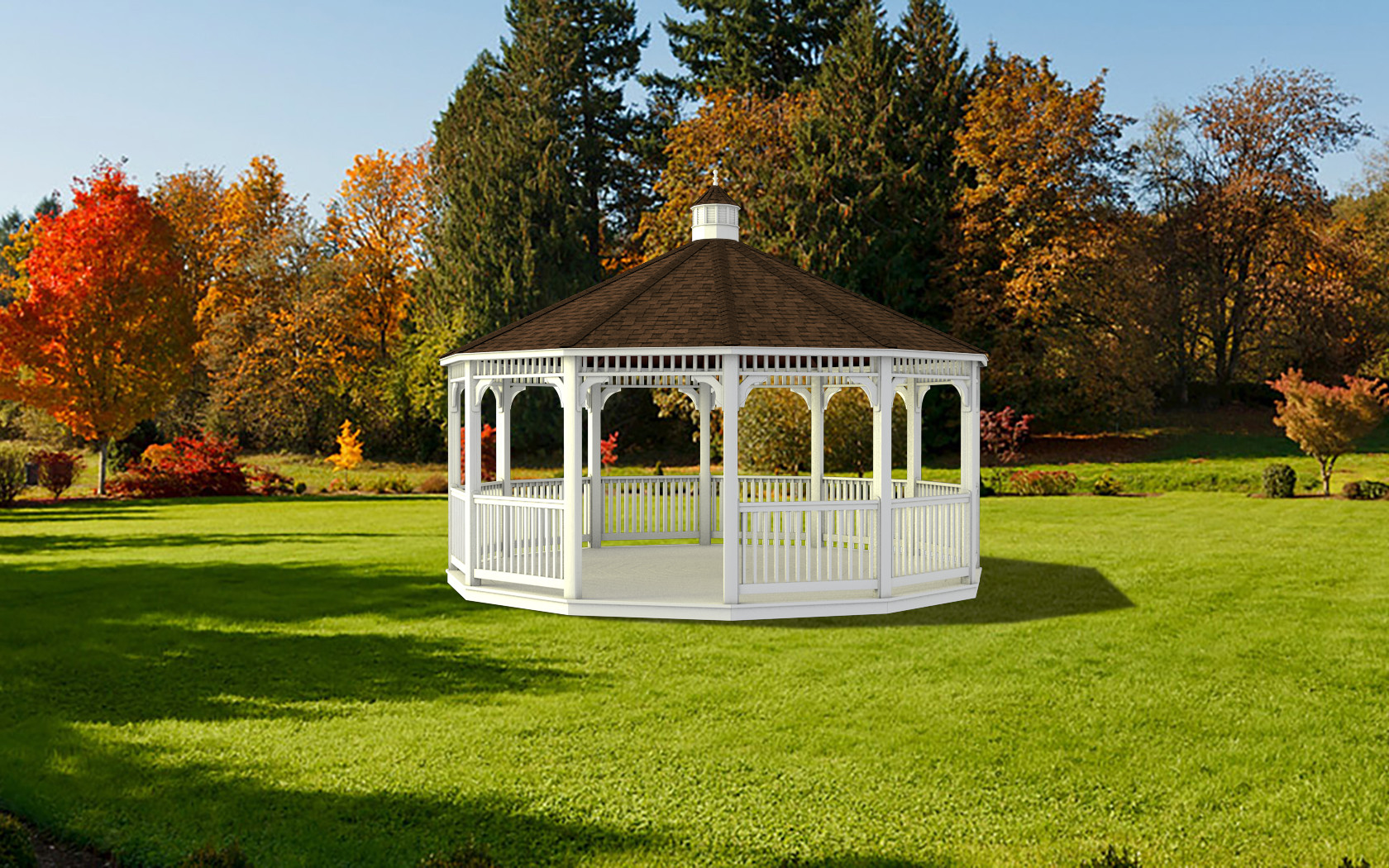The image depicts a well-maintained lawn featuring a white, circular gazebo with a segmented, shingled roof that is mostly brown, contrasted by white trims and rails. A distinctive feature atop the gazebo is a small, white, barn-like structure that also has a brown shingled roof and a weather vane. The gazebo, free of any furniture or arrangements, stands as an open, inviting space in the center of the lawn. Surrounding this pristine area, autumn is in full display, with trees showcasing a kaleidoscope of fall colors—red, yellow, and green. The background includes a row of bushes marking the edge of the lawn before the vibrant trees. The entire scene is bathed in sunlight under a beautiful blue sky, suggesting a perfect, tranquil day.